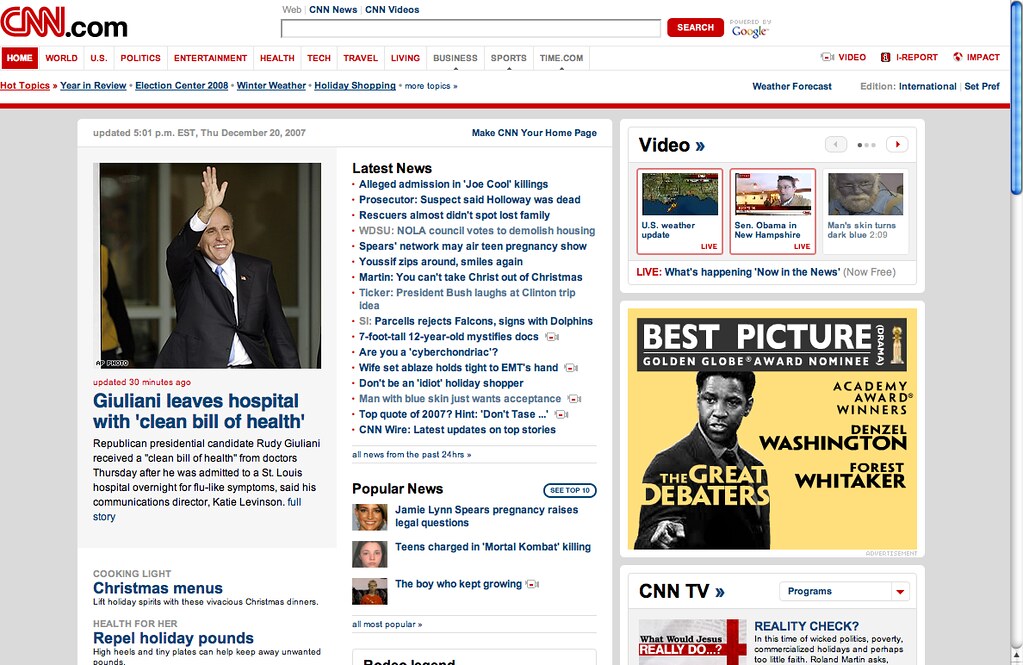The image captures the homepage of CNN's website as viewed on a Mac computer, discernible by the distinctive blue Apple scroll bar on the right. In the top left corner, the site is branded with "cnn.com." Along the very top of the page, a search bar powered by Google is prominently displayed, paired with a red search button for easy querying.

Below this search functionality, a navigational menu spans the page, offering various sections: Home, World News, U.S. Politics, Entertainment, Health, Tech, Travel, Living, Business, and Sports. Adjacent to these, links for 'time.com', 'Video', 'iReport', and 'Impact' invite further exploration.

Directly beneath this menu, a series of prominent topic links appear, featuring "Hot Topics," "Year in Review," "Election Center 2008," "Winter Weather," and "Holiday Shopping," with additional buttons providing access to more topics, weather forecasts, international news, and special sections.

The primary content of the page includes a series of clickable video thumbnails and headlines. Featured here are stories such as:

- "U.S. Weather Update"
- "Senator Obama in New Hampshire"
- "Man's Skin Turns Dark Blue"
- "Live: What's Happening Now in the News"
- "Best Picture for Golden Globe Award Nominee"
- "Denzel Washington: What Would Jesus Really Do?"
- "Reality Check"
- "Jamie Lynn Spears' Pregnancy Raises Legal Questions"
- "Teens Charged in Mortal Combat Killing"
- "The Boy Who Kept Growing."

The most highlighted article focuses on Rudy Giuliani, with the headline "Giuliani Leaves Hospital with Clean Bill of Health." The accompanying text details that Republican presidential candidate Rudy Giuliani was discharged from St. Louis Hospital with a clean bill of health following overnight admission for flu-like symptoms, as confirmed by his communications director, Kate Levinson. A 'Full Story' link offers more details on the event.

Further down the page, additional articles are listed under latest news updates and include a variety of other headlines and stories, such as "Christmas Menus Repel Holiday Pounds," accompanied by myriad other clickable links for the latest news.